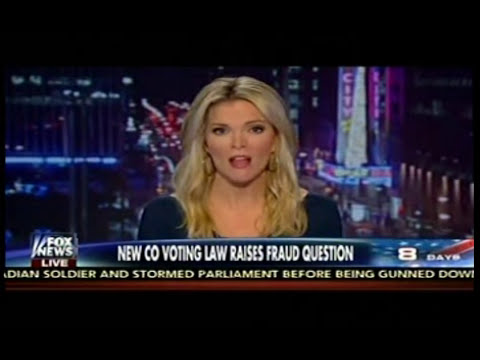This image is a still from a Fox News broadcast, capturing a white female news anchor with blonde hair wearing a blue dress. She is centrally positioned, facing forward with her mouth open as if speaking. Behind her is a nighttime cityscape featuring illuminated buildings and roads, likely utilizing a green screen backdrop. The broadcast features several text overlays: at the top and bottom are horizontal black strips, framing the image. Beneath the anchor, a blue strip with the Fox News Live logo on the left displays the headline "New CO Voting Law Raises Fraud Question" in the center, and "8 days" on the right. Below this, on a black strip, the text reads, "Soldier and stormed parliament before being gunned down." The combined elements of the anchor's appearance, the varied text information, and the urban night backdrop give a clear sense of a dynamic news segment in progress.